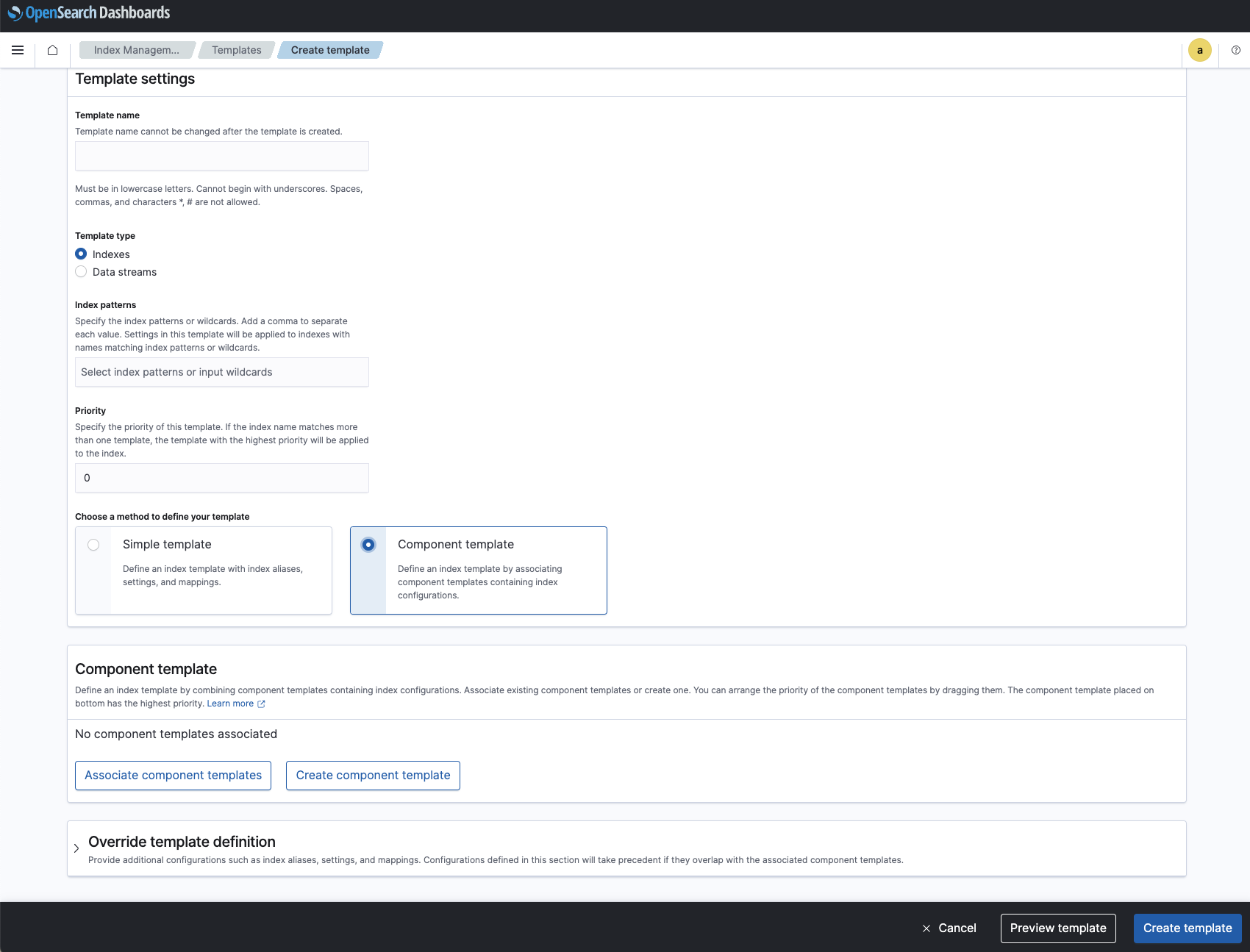Here is a cleaned-up and detailed caption for the screenshot from the OpenSearchDashboards website:

---

This screenshot captures the "Create Templates" section within the OpenSearchDashboards interface. The top header is black, featuring a navigation bar with icons and tabs, including a three-line menu icon, a home icon, and tabs labeled "Index Management," "Templates," and the currently selected tab, "Create Templates."

Starting at the top of the "Create Templates" page, there is a section titled "Template Settings." Below this heading is the "Template Name" field with a text box that includes guidelines stating that the name must only contain lowercase letters and cannot start with underscores. Spaces, commas, and specific characters are not allowed.

Next, the "Template Type" selection offers two options: "Indexes" and "Data Streams," with "Indexes" currently selected. 

Following this, the "Index Patterns" section allows users to specify patterns for the index names, featuring a dropdown menu labeled "Select Index Patterns" or "Info Wildcards."

Further down, the "Priority" section asks users to specify the priority of the template. If an index name matches multiple templates, the template with the highest priority will be applied first. 

There is a "Simple Template" checkbox option that enables users to define an index template with an index alias, settings, and mappings. Adjacent to this is a blue button labeled "Component Template," which allows users to define an index template by associating component templates and coordinating index configurations.

Two white rectangles below this option contain additional settings. One is labeled "Component Template" with a message indicating that no component templates are currently associated. Below this, there are two buttons: "Associate Component Templates" and "Create Component Template."

At the bottom of the page, a section titled "Override Template Definition" is present. 

Finally, the footer of the page features three buttons: "Cancel," "Preview Template," and "Create Template," all positioned within a black footer bar.

---